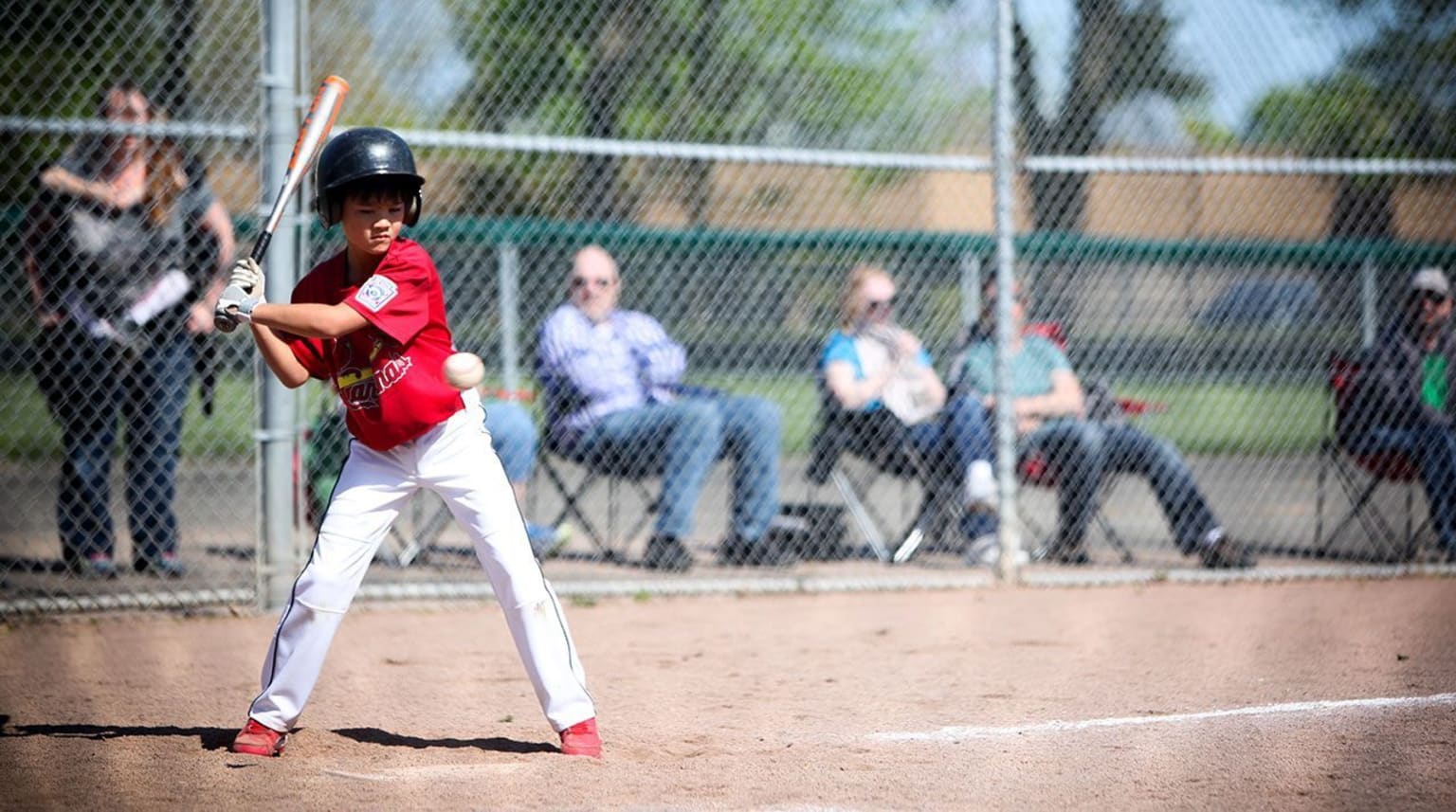This color photograph captures a young Little League baseball player at home plate, preparing to hit a pitched ball that is visible mid-flight, just crossing the plate. The boy, dressed in a red Cardinals jersey, white baseball pants, red sneakers, and a black batting helmet, stands poised with his aluminum baseball bat cocked over his right shoulder. The scene is rich in detail: the dirt ground features a visible third baseline marking, and a large chain-link fence stands behind the boy. Beyond the fence, a group of spectators, likely family members and other supporters, sit in portable folding chairs, with a large woman standing to one side. In the background, the setting includes a brown building, trees, and a clear blue sky, capturing the quintessential feel of a community baseball game.